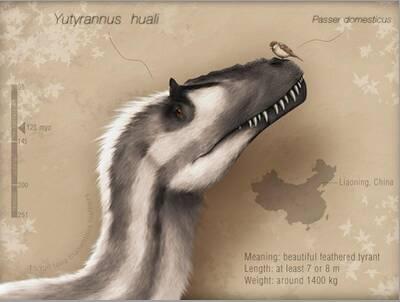This detailed, educational illustration depicts the prehistoric dinosaur Yutyrannus huali, known as the "beautiful feathered tyrant," originating from Liaoning, China. The creature is portrayed with a head resembling the shape of a horse and sharp, exposed teeth. Its body is covered in long, striped fur reminiscent of a dog's or bear's coat, with a striking white stripe running down its head and neck, complemented by dark gray and light tan stripes along its body. A distinctive black snout contrasts the rest of its fur. Perched on the dinosaur's snout is a small bird, Passer domesticus, resembling a common sparrow with a brown back and white chest. The background features a brownish hue with scattered white leaves, and additional details include a map pointing to Liaoning and text specifying the dinosaur's size—about seven to eight meters in length and weighing around 1,400 kilograms. On the left, there's an ambiguous scale labeled "123 NYO" due to blurriness.